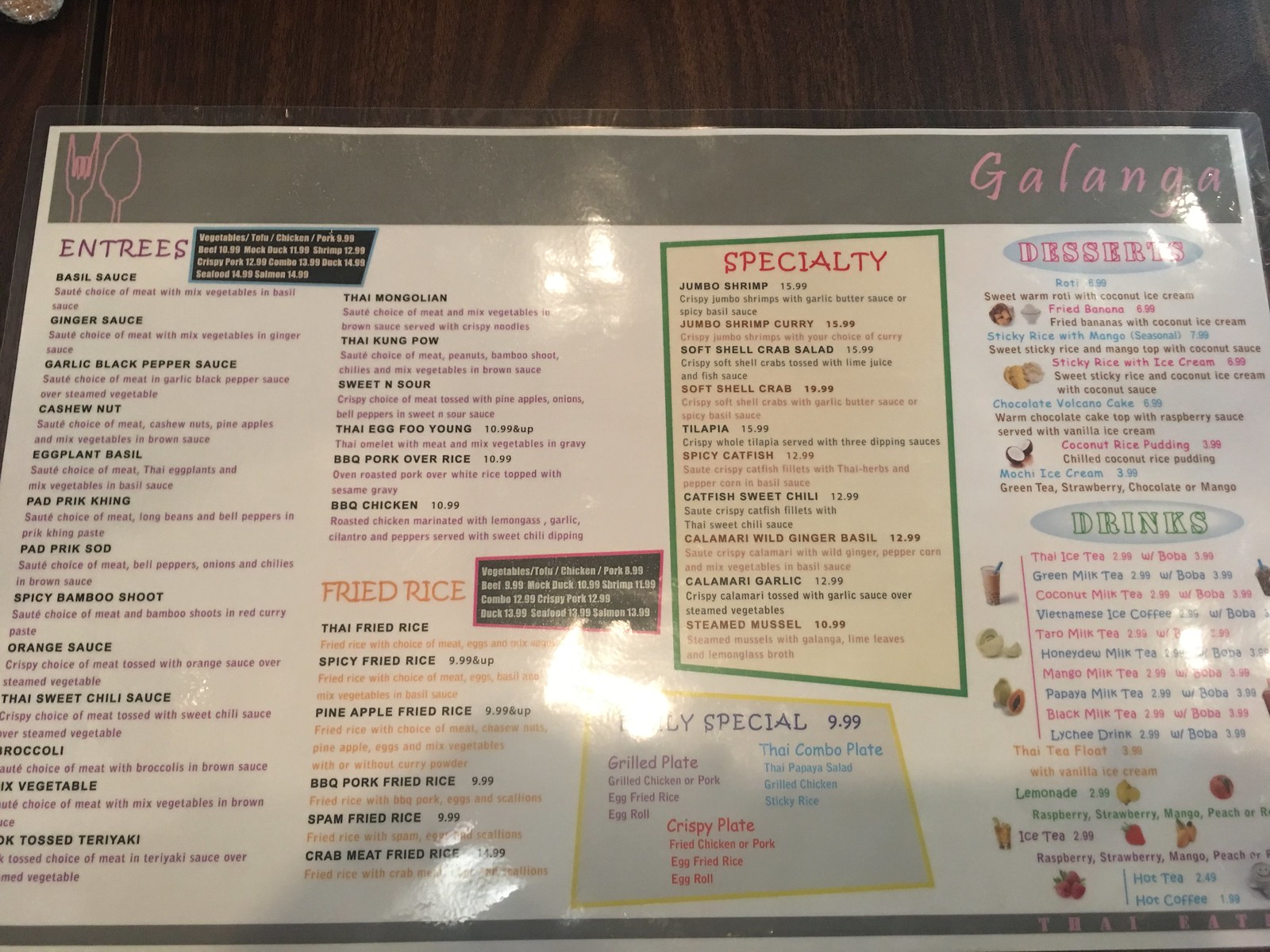The image provides a detailed, top-down bird's-eye view of a laminated rectangular menu set on a wooden table. The perspective suggests a first-person point of view. The menu, laid horizontally, spans across the table, which appears to be composed of two separate wooden sections joined together, indicated by a visible groove about 3-4 cm from the top-left corner. 

In the very top-left corner, a glass container with a ribbed and spiked design slightly protrudes out of the frame. The menu itself features a prominent glare in the middle, reflecting light due to its laminate surface. Additional glares are detectable in the top-right and bottom-right corners. 

The menu is written in English and titled "Galanga," displayed on a brown banner at the top-right, which likely indicates the name of the restaurant. The menu is categorized into several sections: Entrees, Fried Rice, Specialties, Daily Special, Desserts, and Drinks. 

- **Entrees**: Positioned on the left side, this section occupies one and a half columns and offers 17 different options.
- **Fried Rice**: Completes the remaining half of the first column and includes 6 items.
- **Specialties**: Found in a separate green-bordered box with a light green background on the second column, listing 10 options.
- **Daily Special**: Situated below the Specialties, enclosed in a yellow-bordered rectangular box on a grey background. It features three main dishes, each priced at $9.99:
  1. Grilled Plate: Grilled chicken or pork, egg fried rice, egg roll.
  2. Thai Combo Plate: Thai salad, grilled chicken, sticky rice.
  3. Crispy Plate: Fried chicken or pork, egg fried rice, egg roll.
- **Desserts and Drinks**: Located to the right of the Daily Special, the Desserts menu is positioned above the Drinks menu. The Desserts section contains 7 options, and the Drinks section includes 16 selections. 

Menu prices vary from $9 to $20, with drinks and desserts being the most affordable. Notably, the entrees do not display prices next to the items, suggesting that their prices might be listed elsewhere on the menu. Overall, the menu is rich in variety, offering numerous options across all sections.